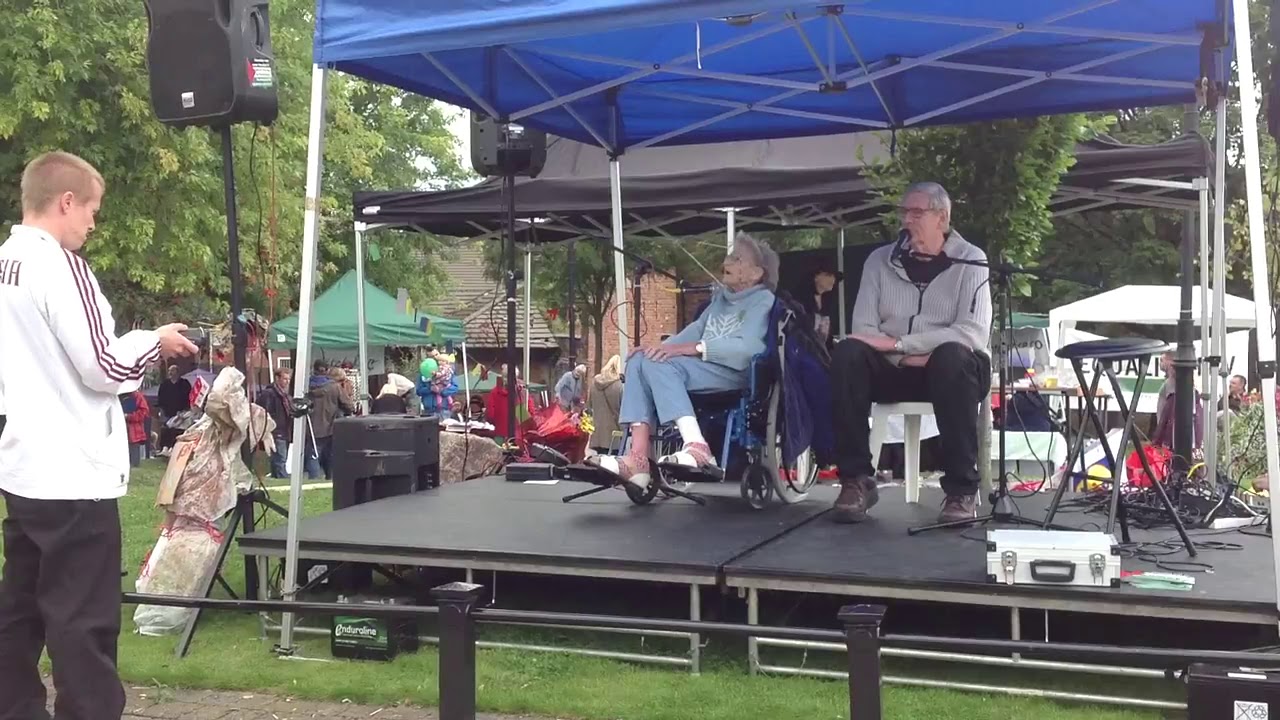The image depicts an outdoor scene at what appears to be a festival or fair, set on a grassy area surrounded by numerous vendor tents and bustling activity. Central to the image is a small black stage with metal framing, topped by a blue tent canopy with four posts at each corner. On the stage, an elderly Caucasian couple is seated: the man on the right in a white plastic chair, dressed in a gray zip-up jacket, black pants, and brown shoes, with a microphone stand positioned at his mouth. Next to him on the left is an elderly woman in a wheelchair, dressed in a powder-blue outfit with a blue sweater and pants, her curly gray hair slightly disheveled as she gazes forward with a relaxed demeanor. To their left stands a middle-aged man in a white sports jumper with black stripes and black pants, holding an object directed at the couple, possibly recording their interaction. In the background, a building and trees frame the scene, with towering speakers on poles flanking the stage, and additional people mingling among the tents, enhancing the lively atmosphere.